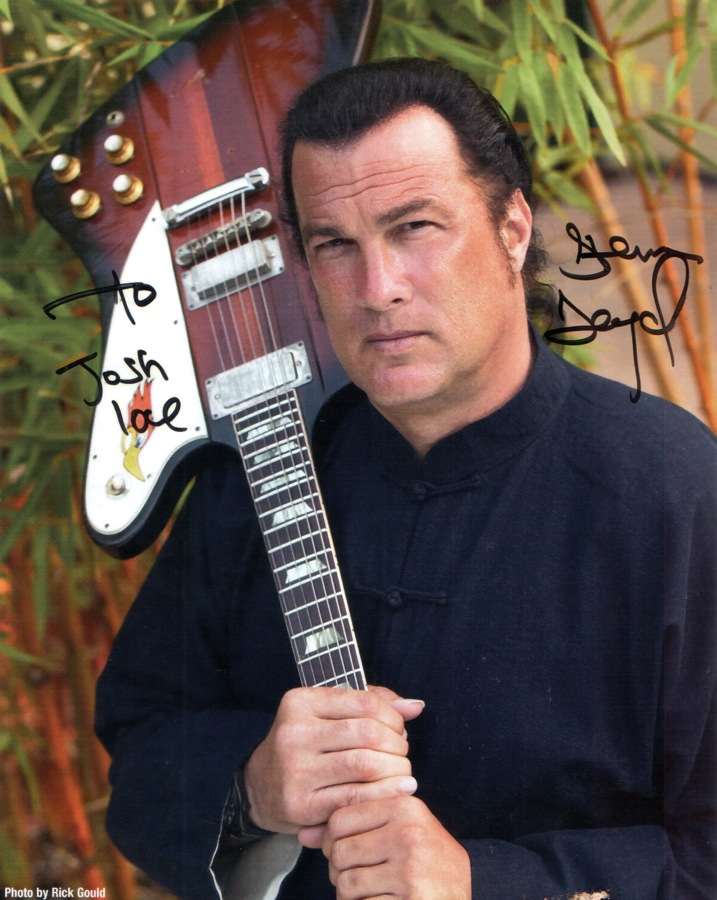The photograph captures a middle-aged Steven Seagal, visibly aged with deep, wavy lines set into his forehead, standing with an electric guitar held by its neck. He wears a dark blue, traditional East Asian-style coat, fastened with knots and strings, and featuring a high collar. Seagal's autograph is scrawled in black marker across the image, with "To Josh Le" written on the left side and "Steven Seagal" on the right. A watermark in the bottom left corner credits "Photo by Rick Gold." The backdrop features indistinct plants, adding a natural element to the scene. The guitar, noticeable for its red base, further accentuates the image's unique composition.